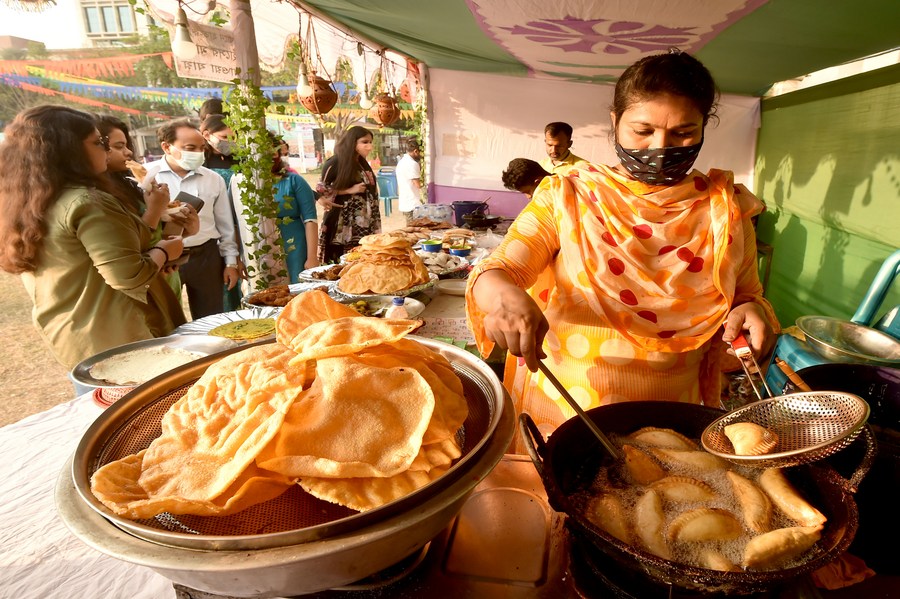The photograph depicts an Indian woman cooking food at an outdoor market, standing under a green canopy. She is dressed in an orange dress adorned with red dots and wears a black and white scarf on her face. The canopy has a light green color with a white section in the middle featuring a purple flower. In the background, the scenery is also light green. The woman is using a metal strainer to spoon out pastries from hot oil in a wok. These pastries resemble mini pot pies. To the left, customers are lining up, likely to purchase the food being prepared. In front of the customers, on a table covered with a white tablecloth, various silver bowls filled with different foods, dips, and tortillas are laid out. Other market participants and decorations, such as green leafy vines around a pole and ribbons with triangular pendants, can be seen throughout the scene. Multiple people in the background are engaged in eating and browsing, contributing to the bustling atmosphere of the market.